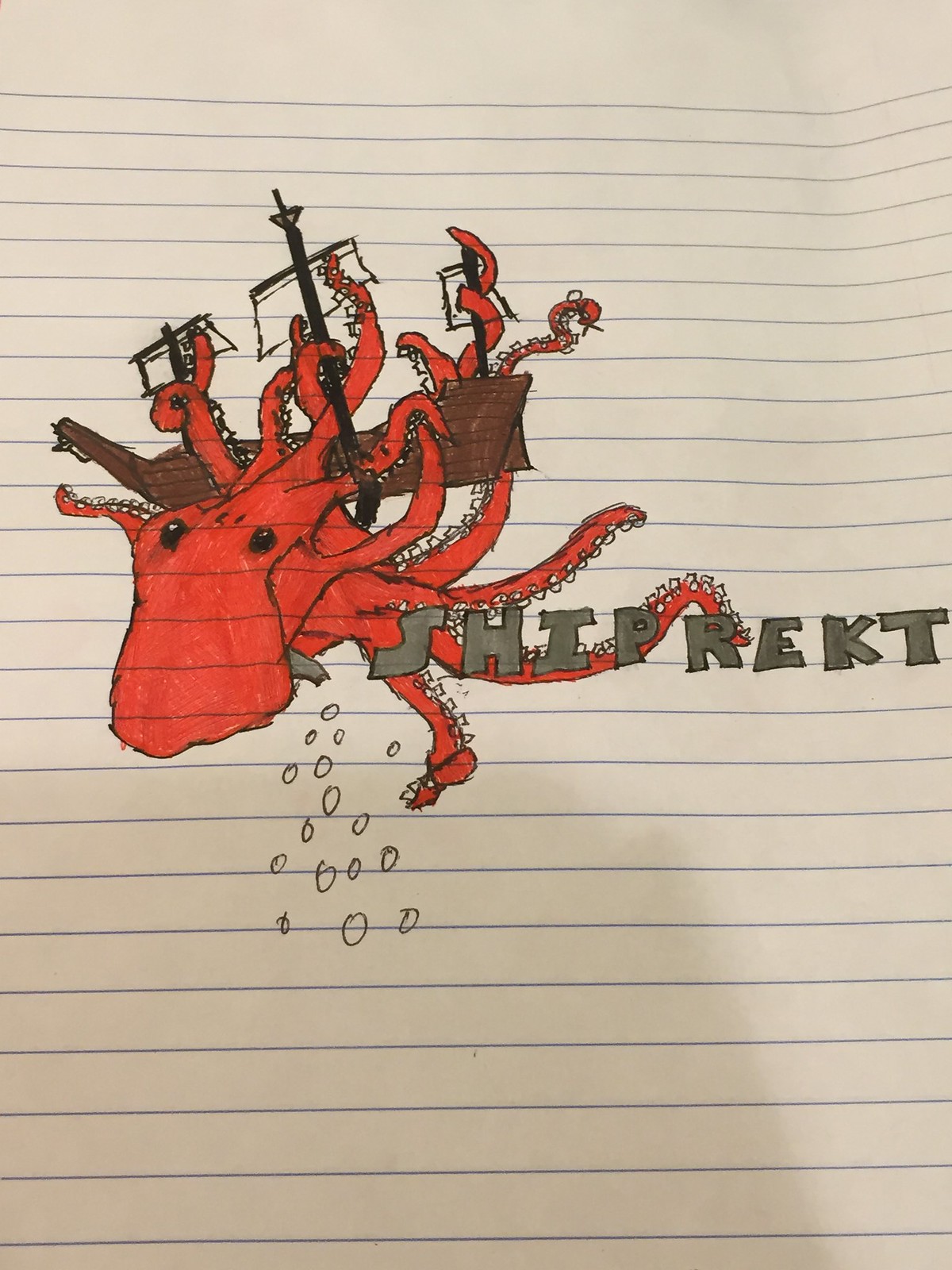This is a color photograph of a detailed, sophisticated line drawing on ruled copybook paper, which has ten thin blue horizontal lines and a wider white margin at the top. The paper appears beige due to poor lighting, and a shadow extends from the left to the bottom part of the picture. Central to the image is an intricate drawing of a red octopus, outlined in black and positioned upside down with numerous tentacles spread out, encompassing an antique-style brown pirate ship. The ship, viewed from the side, has a wooden bottom, three black poles with small rectangular white sails, and an additional long piece extending diagonally to the left of the ship. The octopus’s tentacles are meticulously wrapped around the ship's sails, creating a dramatic visual effect. To the right of the octopus, the word "SHIPREKT" is inscribed in grey block letters. Below the central imagery, several small, imperfectly circular scribbles suggest water droplets.